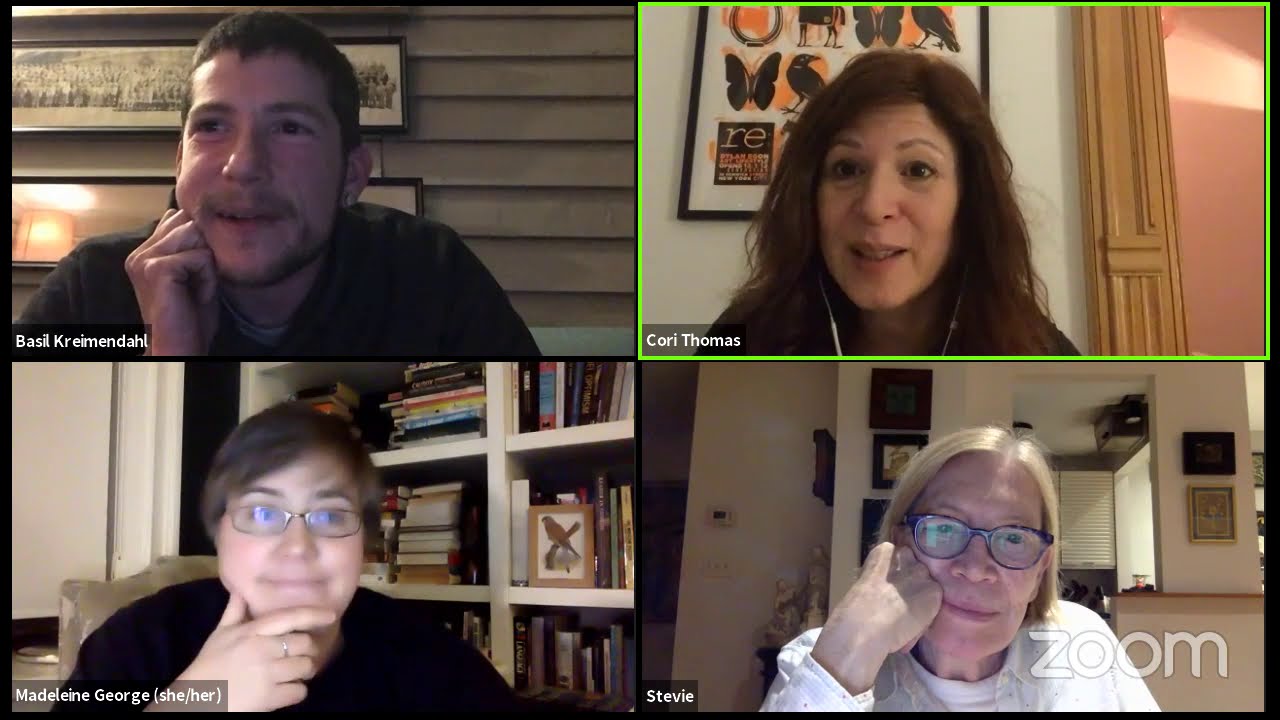This image is a detailed screenshot of a Zoom meeting with four distinct participants, each occupying a quarter of the screen. The Zoom watermark is visible in the bottom right-hand corner. 

In the upper left quadrant, Basil Kremendahl, a man with short brown hair, a mustache, and a goatee, is pictured against the wall of his home, with some pictures visible in the background. He is leaning forward with his hand under his chin.

The upper right quadrant features Corey Thomas, a woman with long brown hair and in-ear headphones whose cord is visible. She is positioned against the wall of what appears to be a bedroom, with a photo frame located over a doorway in the background.

In the lower left quadrant, Madeline George (she/her) appears. She wears glasses and has short brown hair, and she is in front of a background filled with bookshelves. She is resting her chin on her hand.

The bottom right quadrant shows Stevie, an older woman with straight blonde hair and glasses, wearing a white sweatshirt. She is also resting her hand on her face, and behind her, a setting that may resemble a dining room is partially visible.